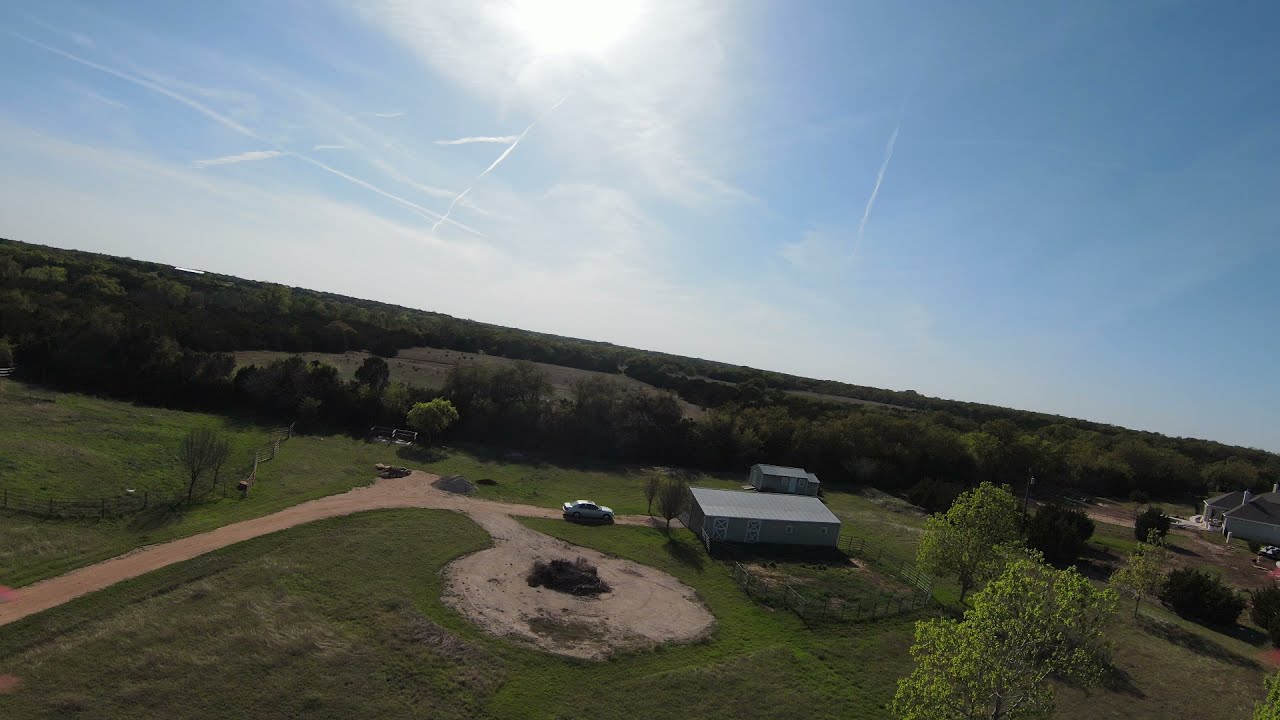The image presents an aerial, slightly angled perspective of a pastoral country property. In the center of the image, a blue-gray house is slightly below the dead center. To its left is a circular, dirt driveway where a white four-door sedan is parked. The driveway extends outward from the frame on the left side. Adjacent to the house, scattered trees dot the grassy landscape, giving way to expansive fields visible behind the property.

A second building, with a tan roof, can be seen on the right side of the image, partially cut off by the frame. It's suggested that this might be the neighbor's house. Both buildings feature white-trimmed doors. The sky takes up roughly the top half of the image, painted in shades of blue and white with scattered clouds and visible contrails. The bright sun shines at the top center, creating a lens flare that draws the eye. The whole scene is bathed in natural light, highlighting the rich brown of the roads, the lush green of the grass and trees, and the expansive open field behind the houses.